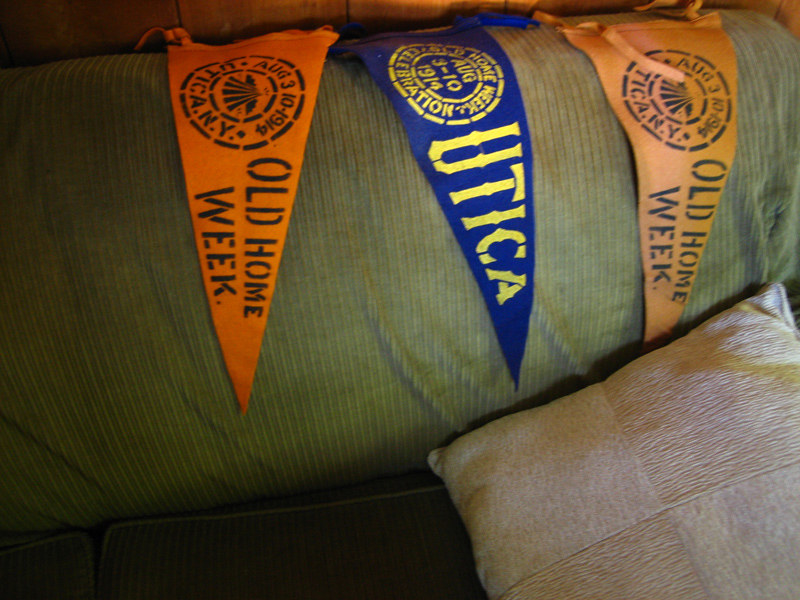The image showcases three triangular pennants draped over the dark green cushion of a couch, which features a decorative pillow in front. Each pennant commemorates "Old Home Week," an event held from August 3 to 10, 1914, in Utica. The pennants are arrayed in descending order: the top one is a faded orange with black lettering, the middle one is blue with gold letters spelling "UTICA," and the bottom one is a bright orange with clear black lettering. They all share the same details about the event date and location, emphasizing their historical significance. The couch and the visually distinctive arrangement of pennants make it appear as if showcasing these nostalgic memorabilia, possibly for an online marketplace.